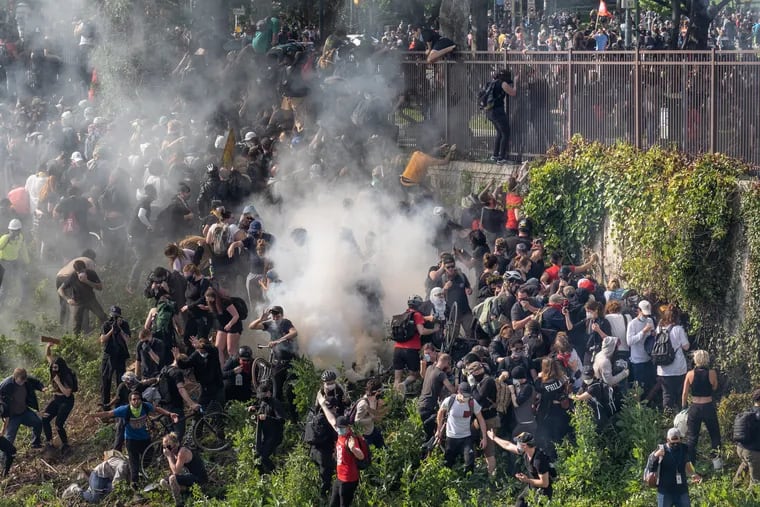The image depicts a chaotic protest scene with a palpable sense of anarchy. In the foreground, a large crowd of people, diverse in age and attire—mostly t-shirts, dark pants, red shirts, black shorts, white t-shirts, and sleeveless tops—are seen attempting to climb over a tall metal fence above a substantial stone wall. The area is enveloped in thick white smoke, suggesting that tear gas has been deployed, likely by police, to disperse the gathering. Some individuals can be seen wearing masks over their mouths and stopping to cover their eyes from the tear gas. Bicycles are scattered amidst the crowd, and the lower left of the scene features a grassy hill leading up to the stone wall. The chaos continues beyond the fence, where another massive group of people is densely packed. The atmosphere is intense and frenzied, with people in various states of panic, and the scenery dominated by green, vine-like vegetation interspersed with the unsettling urgency of the protest.